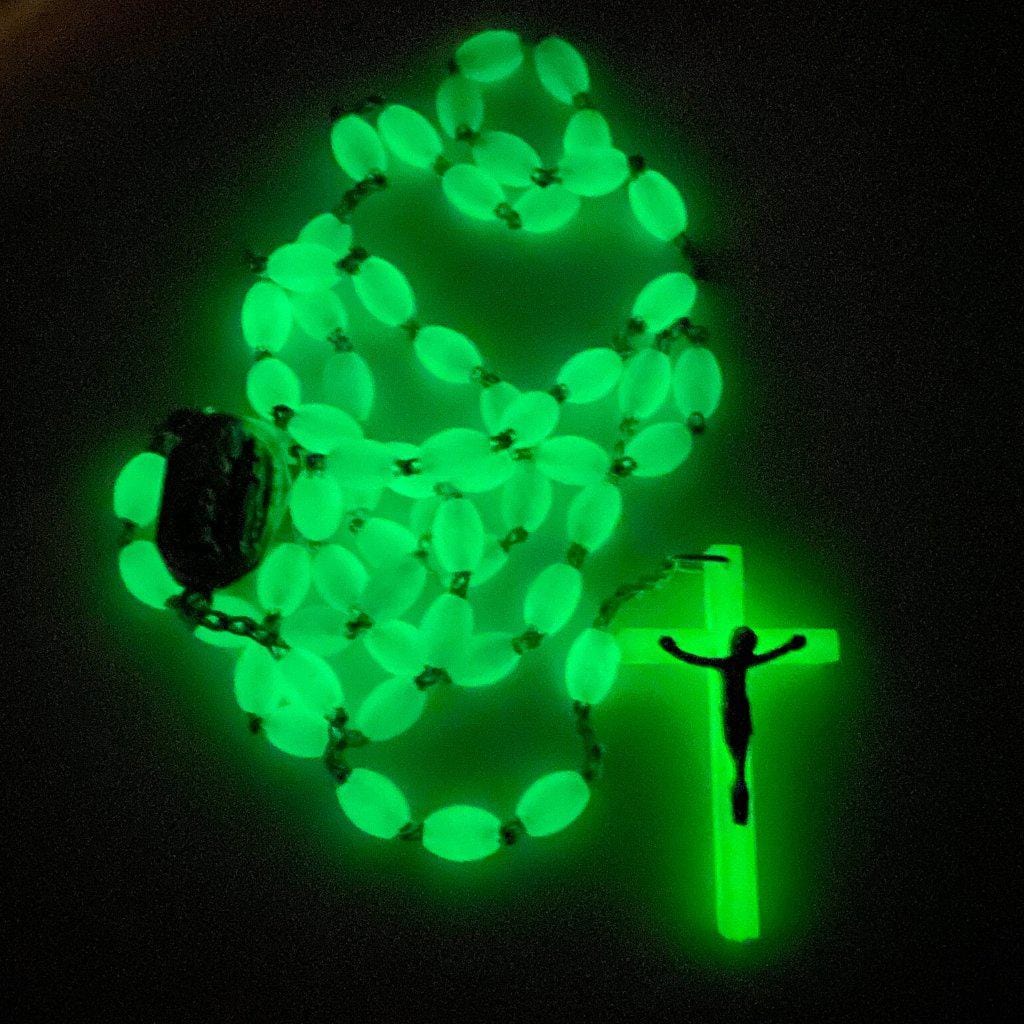In this image, a necklace featuring a cross is prominently displayed, set against a completely black background. The necklace appears to have white beads that form the chain, though under the illumination, these beads glow a bright lime green. The centerpiece of the necklace is a cross that vividly glows a very bright green, with the silhouette of Jesus on the cross rendered in stark black. This glow-in-the-dark effect gives the entire piece a luminescent, almost night-vision appearance, making the beads, chain, and cross appear as if bathed in neon green light. Despite the darkness obscuring fine details, the overall ethereal and radiant quality of the necklace and cross is unmistakable.